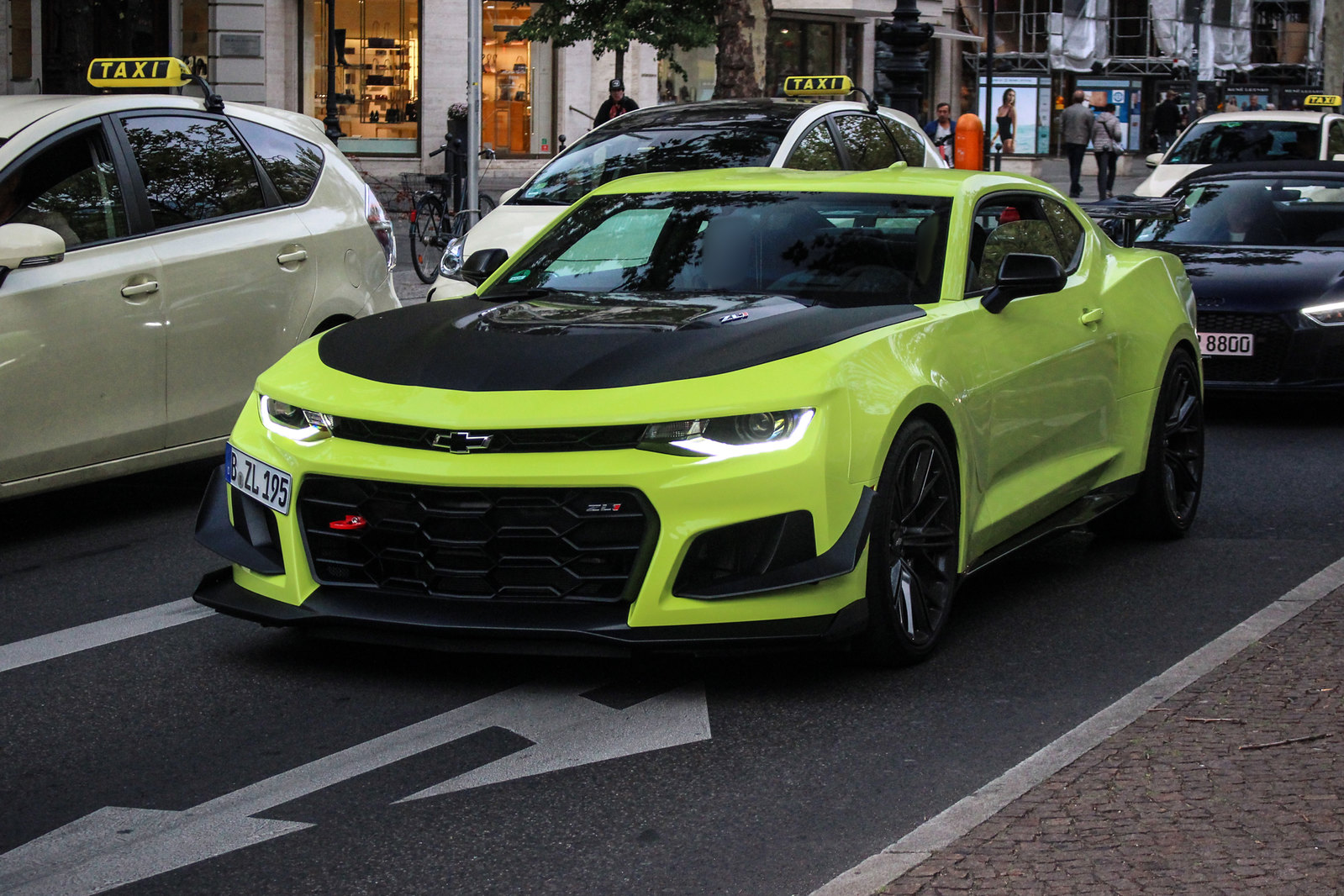A vibrant lime green Chevrolet sports car, possibly a Camaro, with a black hood, black trim, and black rims, dominates the foreground of this bustling city street scene. The car is positioned in a left turn lane, indicated by a white arrow on the pavement showing both left-turn and straight-ahead options. Its distinctive Chevy logo is visible on the front, along with a license plate reading BZL 195. The setting appears to be a European city, likely the UK, due to the format of the license plates and the presence of several white taxis marked with the word "Taxi" on their roofs. Behind the neon-colored Chevrolet, a black car with the license plate BB00 is seen. On the left side of the image, three white taxis create a line, contributing to the busy urban atmosphere. In the background, pedestrians walk along the sidewalk, flanked by various stores and advertisements that lend a lively character to the downtown area. The overall scene is captured in daylight, adding to the vibrant energy of the city street.